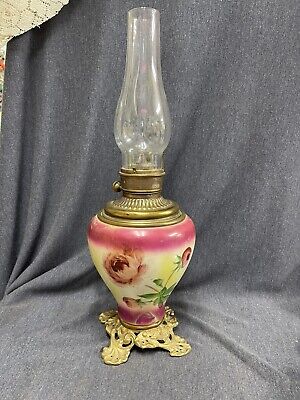This image portrays a vintage hurricane oil lamp set against a gray fabric background, with a hint of white lace visible in the top left corner. The lamp features a decorative gold or brass base designed with elaborate floral patterns and supported by four ornate feet. The body of the lamp is a round ceramic vase, adorned with a thick pink stripe at the top and bottom. The central section of the vase is white, showcasing delicate pink roses and green leaves. Above the ceramic section, a tarnished gold or brass rim transitions into a clear glass chimney. This glass chimney is bulbous at the lower part and narrows into a cylindrical shape at the top, designed to protect the flame. A small twisty knob for adjusting the wick is also present on the back side of the lamp.